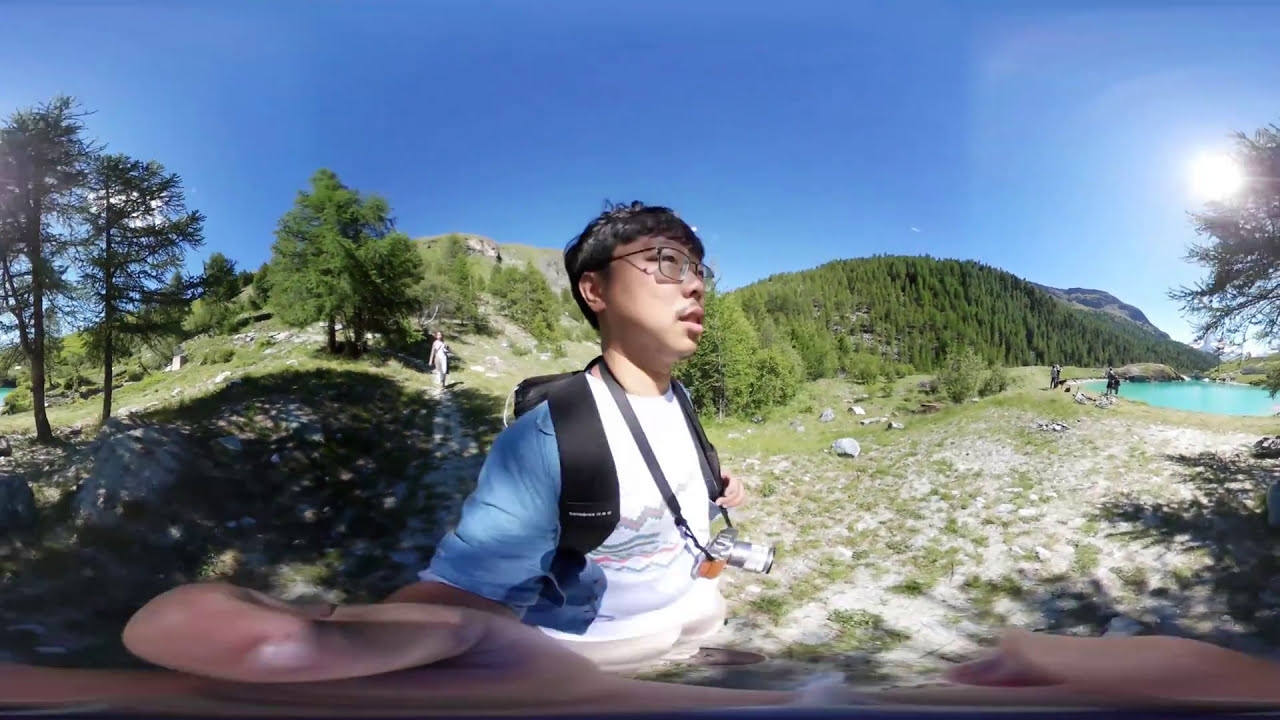In this detailed 360-degree image, we see a young Asian male with curly black hair and glasses, standing centrally in a scenic outdoor setting, likely taking a wide selfie. He wears a white t-shirt with an indistinct design and has a camera around his neck and a backpack on his back. His finger partially intrudes into the shot as he squints slightly with his mouth partially open. Surrounding him is a rugged, uneven rocky terrain dotted with scrubby greenery and small trees. To the right, there is a distinct turquoise-blue thermal pool or swimming hole in the distance. Behind him, a walking path extends into the background, where another person can be seen approaching the camera. The entire scene is bathed in the light of a setting sun, creating a picturesque twilight atmosphere with a colorful palette that includes hues of blue, gray, white, green, tan, orange, and pink. The sky above is clear, further enhancing the natural, serene beauty of the valley with sandy ground, scattered plants, and patches of grass. Pine trees can be seen on a hill to the left, completing this immersive and tranquil landscape.